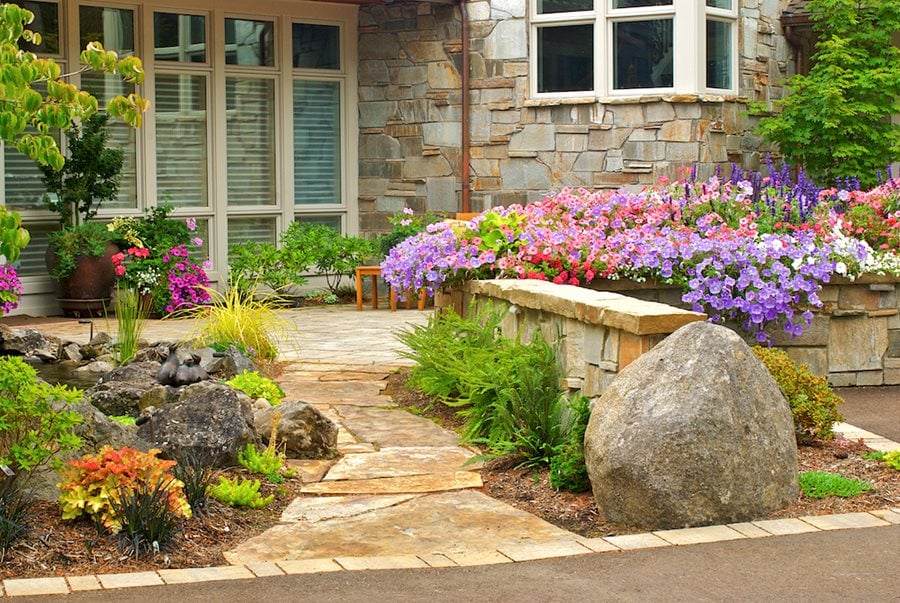This image captures the charming front entrance of a house, beautifully framed by a stone pathway leading up to the home from a stony driveway. The pathway is bordered by lush, diverse plant life, with an array of vibrant flowers adding a splash of color. On the right side, a variety of purple, pink, and deep pinkish-red flowers flourish atop a stone barricade that separates the driveway from the path. The pathway itself is surrounded by more rocks and potted plants, enhancing the inviting atmosphere. The house features several windows in various rectangular and square shapes, each adorned with white blinds. Additionally, the top right section of the house displays more windows, hinting at a second story or additional rooms. A mature tree in the background on the right side completes the picturesque scene, adding a touch of natural elegance to the home.